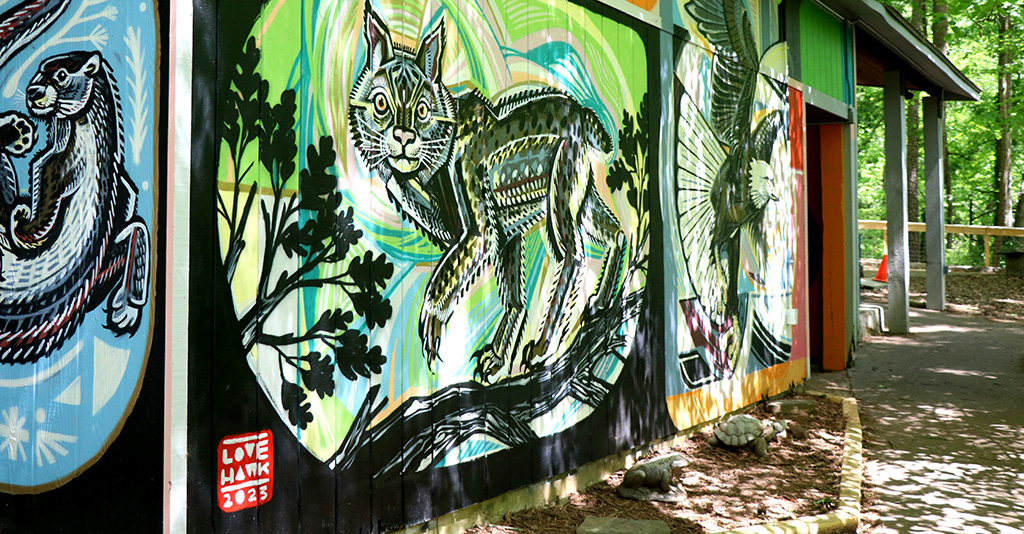This photograph captures the side wall of a single-story building adorned with a vibrant mural, set against an outdoor backdrop of tall, leafy trees. The mural spans multiple square sections, each featuring a different animal painted in a unique style, combining lifelike and abstract elements. The most prominent part of the mural showcases a cat in profile, accentuated with yellow and green squiggle patterns on its fur, set against a variety of colored backgrounds. To the left of the cat, a tree branch with leaves adds a natural element, while the bottom left corner is marked with the text "Love Hawk 2023." Adjacent to the cat mural, an illustration of a bald eagle in flight occupies its own square section. Another mural nearby portrays a stylized sea otter against a blue backdrop dotted with white triangles and stars. A wooden porch with an overhanging gabled roof, supported by two gray pillars, extends from the building, casting shadows across the sandy, shaded ground where ceramic or perhaps real turtles can be seen among other small animal sculptures.